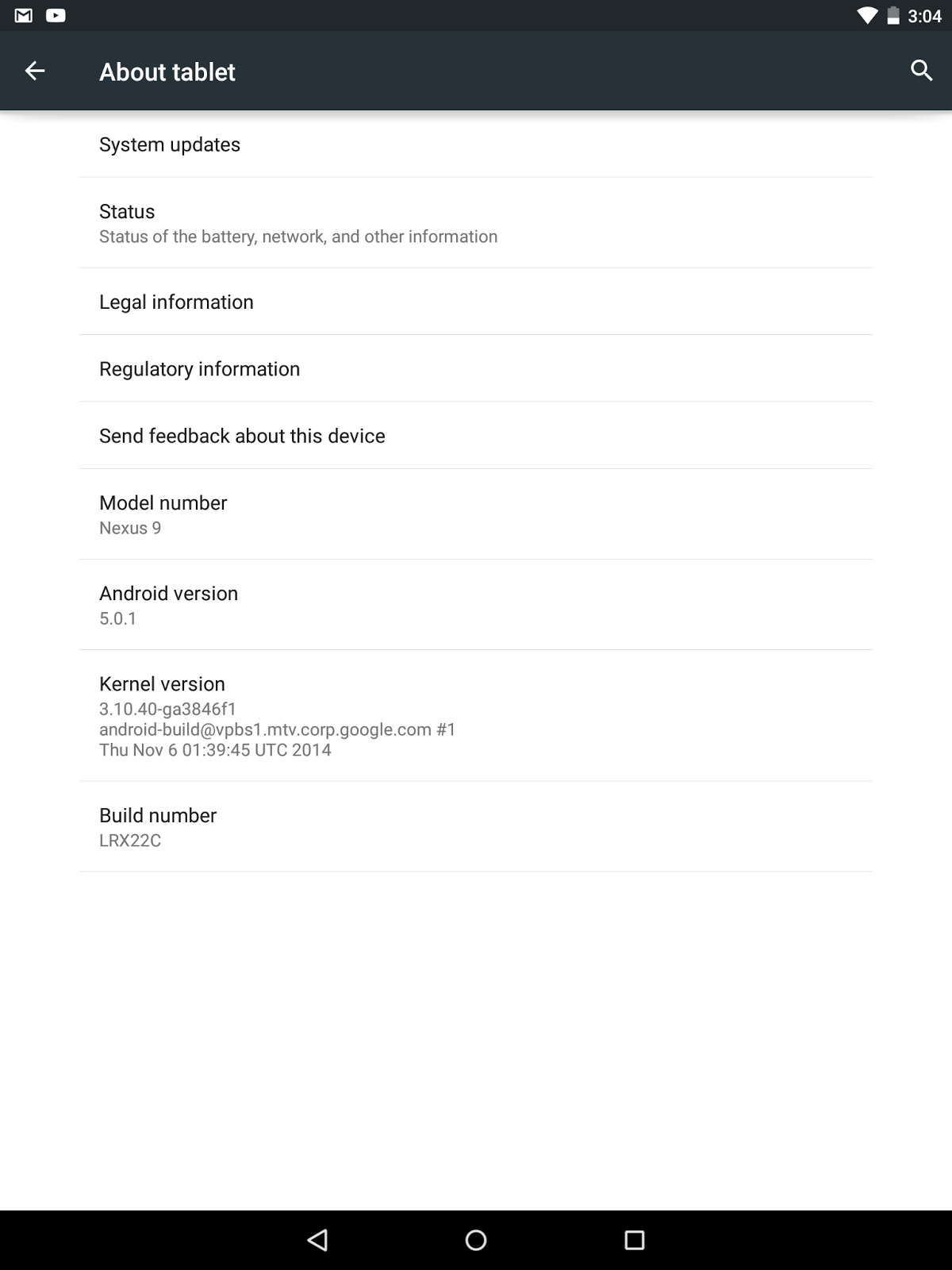This image showcases a web page viewed on a tablet, displaying key information relating to the device's system settings. Starting from the top left, there is a Gmail icon resembling an envelope with a black "M" shape, a YouTube notification icon represented as a white square with a right-facing black triangle, followed by a full white Wi-Fi signal icon. To the right, the battery indicator shows approximately one-third capacity, and the time is displayed as 15:04 (military time), all on a black status bar. 

Below the status bar, a dark blue header features a prominent white left-pointing arrow alongside the text "About tablet," indicating that the screenshot is taken from a tablet device. On the right of this header is a white magnifying glass icon. 

The main content of the web page is set against a white background, displaying system settings in bold black text. Each section heading is clearly demarcated in bold type, with descriptive details underneath in regular black text. The sections include:

- **System updates**
- **Status:** Details about the battery status, network, and other information.
- **Legal information**
- **Regulatory information**
- **Send feedback about this device**
- **Model number:** Nexus 9
- **Android version:** 5.0.1
- **Kindle version:** 3.10.40-GA3846F1
- **Build info:** Android-build at vpbs1.mtv.corp.google.com, number one, Thursday, November 6th, 01:39:45 UTC 2014
- **Build number:** LRX22C

At the bottom of the screen, the navigation bezel is black with a white left-pointing arrow on the left side, a white circle in the middle, and a white square on the right side.